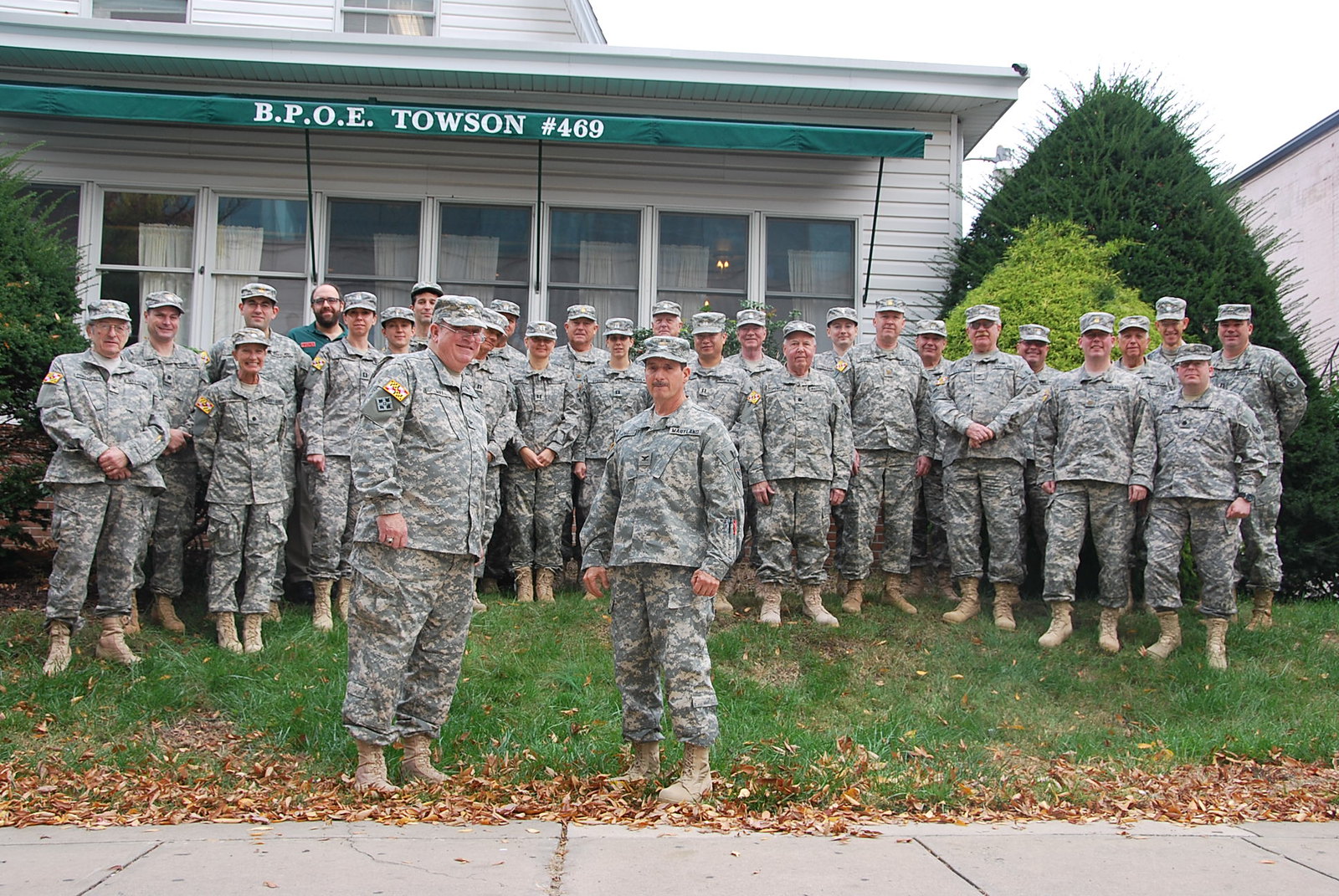In front of a white, two-story building with large glass windows and a green canopy inscribed with "B.P.O.E. Towson 469," stands a diverse group of soldiers and a few women, all facing the camera. They are dressed in camouflage fatigue uniforms with chromophore colors akin to nature, including hats, and military patches on their right arms. The two rows of soldiers, mostly older men, have two individuals in the forefront smiling directly at the camera. They stand on a lawn strewn with orange and yellow fallen leaves, bordered by a concrete sidewalk. Behind them, large, dark green bushes, including a cone-shaped one with lighter green at its base, add to the scene's backdrop.